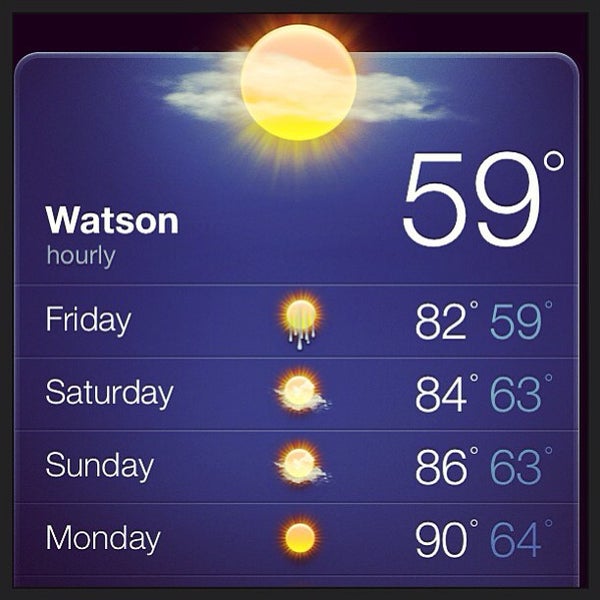The image features a weather forecast divided into four sections, each representing a different day. The edges of the forecast are black, framing the vivid blue sky with scattered clouds in the background. The first section for Friday shows a bright sun with rays shining intensely, indicating a high of 82°F and a low of 59°F. Saturday's section also features the sun, partially obscured by clouds, forecasting a high of 84°F and a low of 63°F. On Sunday, the sun is clearly visible again, with a high of 86°F and a low of 63°F. The final section, Monday, displays a radiant sun with temperatures peaking at 90°F and dipping to 64°F. The dividing lines between the days are semi-transparent, subtly distinguishing each section. The names "Watson" and "Harley" appear within the frame, and the overall aesthetic is clean and informative, with distinct visuals and temperature readings for each day.